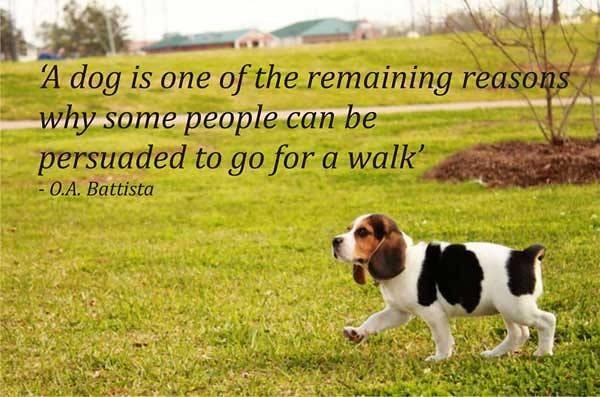The image presents an inspiring and somewhat humorous scene, reminiscent of a greeting card or poster. It features a lush, green park with a grassy expanse and a cement sidewalk running from left to right. In the distance, the slightly blurry backdrop reveals some homes or possibly a school with a green roof, nestled among a few trees, including a tree emerging from a patch of pine straw. The sky appears overcast, adding a calm ambiance to the scene.

Dominating the bottom right corner is an adorable beagle puppy, captured in a side profile as it confidently strides towards the left. The puppy has a charming brown face, droopy ears, a black nose, and its body is a mix of black patches on a primarily white coat. There are no signs of an owner, leash, or collar, evoking a sense of carefree exploration.

Overlaying this picturesque scene is a quote by O.A. Batista: "A dog is one of the remaining reasons why some people can be persuaded to go for a walk." This text adds a touch of snarky wisdom, highlighting the endearing power of dogs to motivate their owners to enjoy the simple pleasure of a walk.